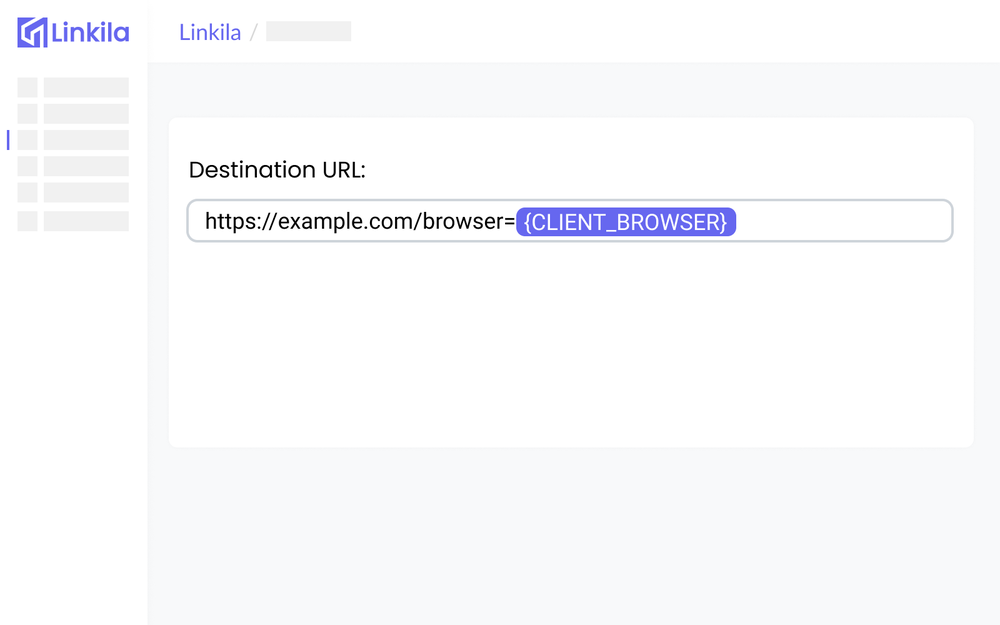This image is a partial screenshot of a webpage with a predominantly white background. In the upper left corner, the name "Linkila" is displayed in a lavender font, accompanied to its left by the company's logo—a lavender square featuring a stylized design where the right side resembles an upside-down "L". To the right of this logo and name, "Linkila" is also written again, this time in a lighter and thinner font.

Positioned slightly to the right of the logo, in the center-left section of the image, the text "Destination URL" appears in a dark gray font. Below this heading, there is a long rectangular field outlined in light gray that contains a web URL: "https://example.com/browser=". Within this URL, a segment is highlighted in lavender and features bold, white capital letters enclosed in brackets: "[client_browser]".

Additionally, along the left side of the page, beneath the "Linkila" name and logo, there is a sidebar composed of six very light gray rectangular placeholders, stacked vertically. This ends the visual details evident in the screenshot.